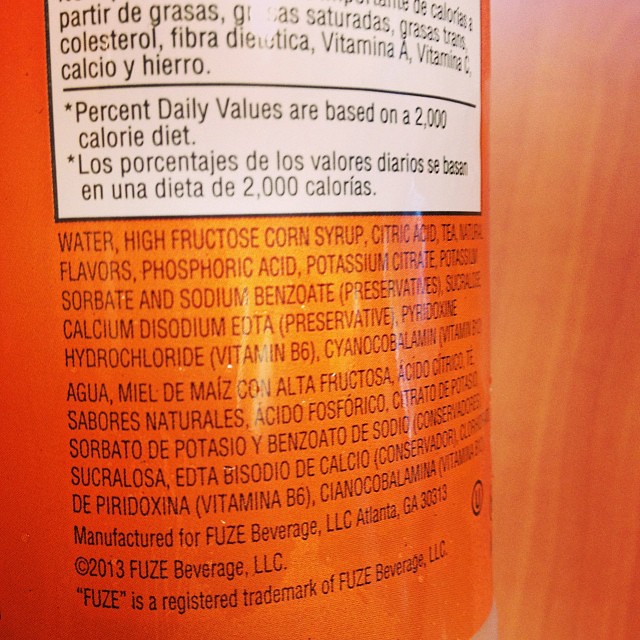This detailed close-up photograph captures the back of a tall, orange can of Fuze beverage being held over a light-colored wood table. The can's label features a prominent yellow and orange gradient background, with the center section appearing lighter. Central to the image is the comprehensive ingredients panel written in small, black text. Below the ingredients in English, the same list is repeated in Spanish. Further down, the text indicates that the beverage is manufactured for Fuze Beverage LLC, Atlanta, Georgia with a trademark note. Above the ingredients section, a white Nutrition Facts panel details the daily values based on a 2000-calorie diet, followed by a Spanish translation. The right side of the image also shows partial reflections of some lights on the can’s shiny surface. An additional detail includes a small ‘U for you’ logo positioned on the right side of the can.